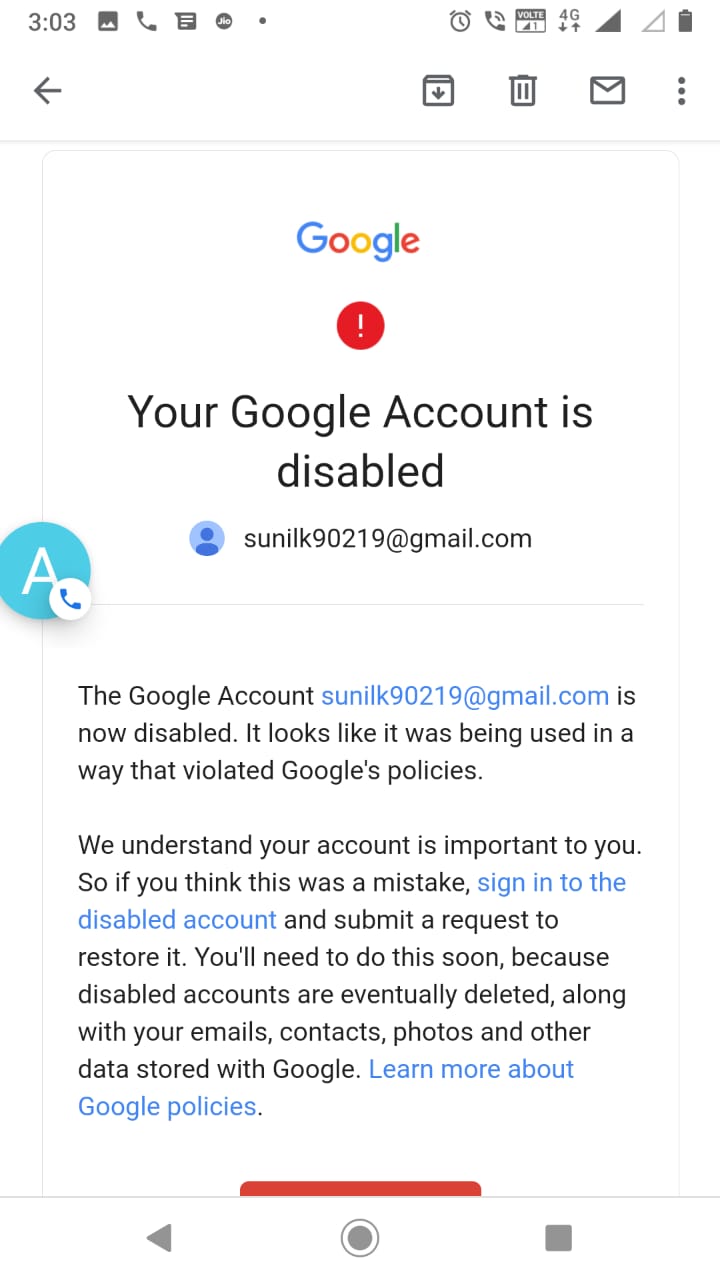This image is a screenshot captured on a smartphone, showcasing a notification indicating that a Google account has been disabled. The screenshot is dominated by a clean, white background. At the top left corner, the time "3:03" is displayed in black text. Adjacent to it, a series of icons including a picture icon, phone icon, message icon, and an indiscernible circular icon appear. Next to them is a small dot. On the right side of the top bar, a nearly full battery icon (approximately 90%) is visible, followed by a filled WiFi icon, a 4G icon with up and down arrows underneath it, a "VOLTE" icon on a grey background, and a ringer icon. The clock icon is next to a back arrow on the left side, and to the right are three vertical dots, suggesting a menu. 

Further down, there's the classic Google logo in its colorful design, followed by a red circle with a white exclamation mark. Beneath that, bold black text declares, "Your Google account is disabled." A light blue and dark blue background frames an account icon. Below that, an email address is listed next to a large blue circle containing a white "A" with a small white circle at the bottom right corner featuring a blue phone. Three lines of information explain the account's disabled status, followed by eight lines of instructions on restoring the account if the disablement was a mistake.

Towards the bottom center, a thin grey line spans horizontally. At the very bottom left, there's a grey triangle pointing left. The bottom center hosts a grey circle with a white border, and on the right, a grey square completes the bottom icon arrangement.